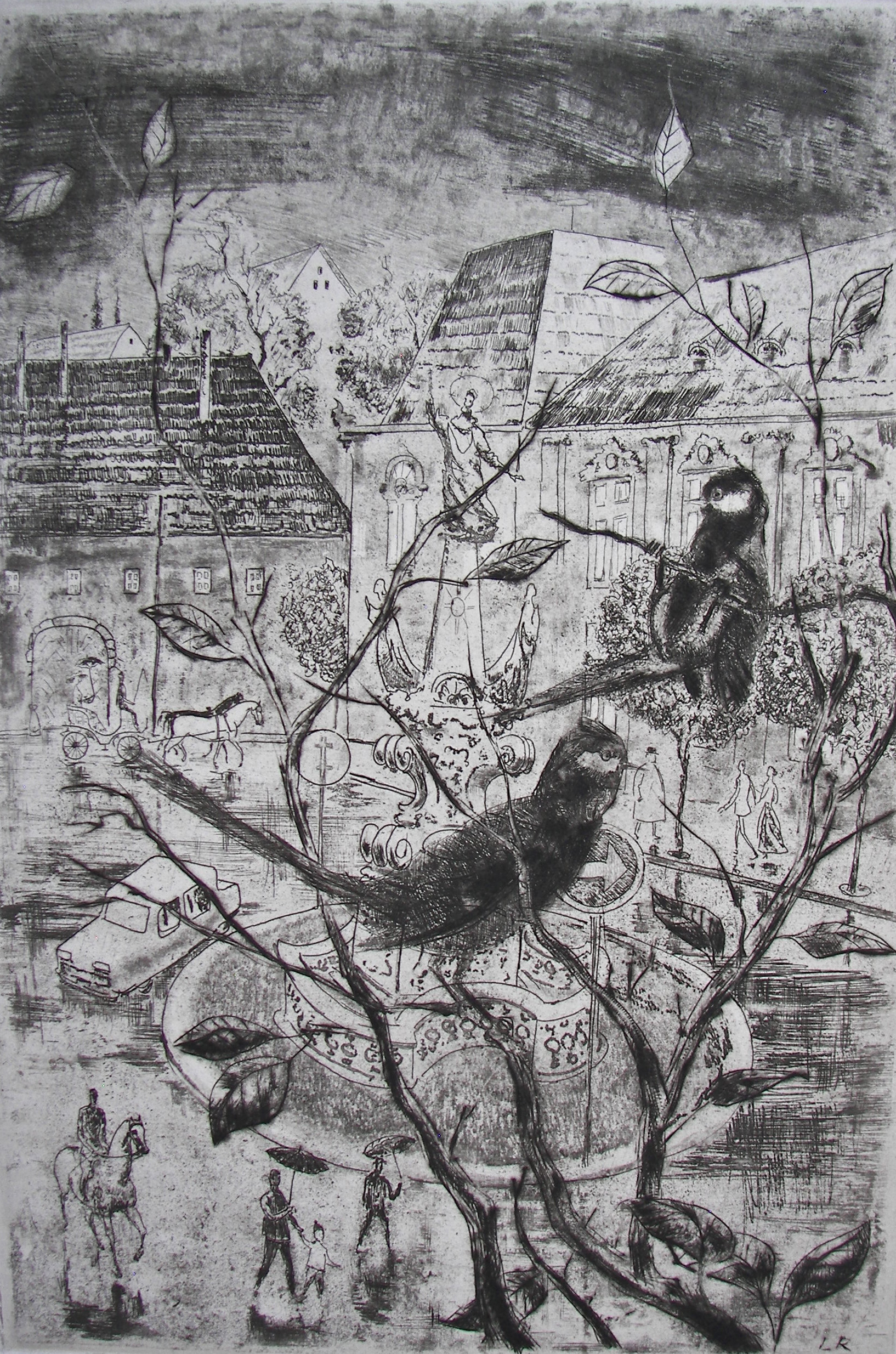The image is a detailed pencil or charcoal drawing of a town on a rainy, overcast day, rendered entirely in black, white, and various shades of gray. At the center of the scene is a roundabout, featuring a large fountain or statue as its focal point. The roundabout is encircled by several cars and pedestrians, all moving in a counterclockwise direction, guided by a directional arrow. Among the figures, a rider on horseback is visible in the lower left-hand corner, alongside two people walking under umbrellas, one of whom is holding a child's hand. The background includes additional buildings and a carriage pulled by two horses. Dominating the foreground are tree branches with sparse leaves, upon which two dark-feathered birds are perched, observing the town below. The sky is heavily overcast with streaks of dark gray and black, contributing to the stormy, rainy atmosphere.